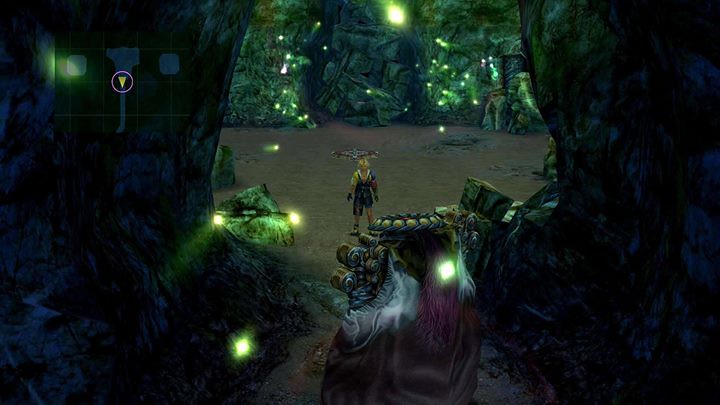In this horizontally-oriented rectangular image, we are immersed in a scene that resembles a moment from a video game set in a magical or futuristic world. The edges of the scene are shrouded in darkness, giving the impression that we are peering out from within a cave. At the center of the image, there is an irregularly-shaped but generally circular opening through which we can see the main subject—a young man standing on a flat patch of brown dirt. Flanking him are several large boulders.

The young man, though not in close view, appears to have blonde hair and is dressed in a light-colored shirt paired with a vest and shorts. Beyond him stretches a vibrant expanse of greenery. The terrain transitions from the dirt ground to either vegetation or rocks that emit a greenish hue, though the details are somewhat blurred, making it challenging to discern the exact nature of this element.

In the upper left corner of the image, there is an icon that resembles a weapon, signified by a yellow triangle inside a circle, which is highlighted, adding to the overall mysterious and adventurous atmosphere of the scene.